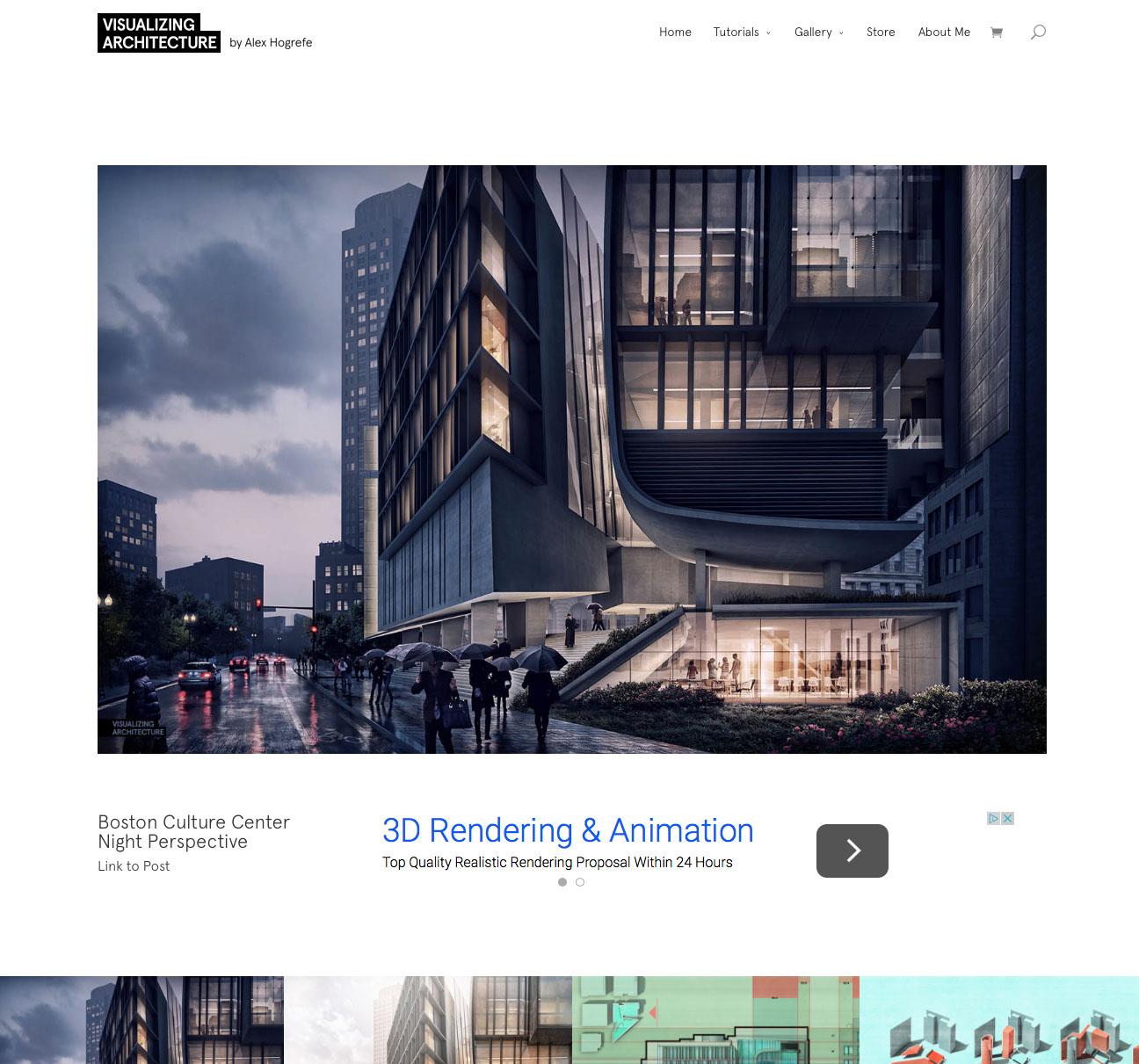Screenshot of a professional architecture website. The top section displays a white background with a black header on the left side reading "Visualizing Architecture" in white text. Adjacent to the header, on the white section, is the byline "By Alex Hogrefe". On the right side, a navigation bar offers options: Home, Tutorials, Gallery, Store, About Me, Shopping Cart, and a magnifying glass icon for search functionality.

Below the header is a vivid, modern cityscape image, depicting a rainy scene with multi-story buildings, pedestrians with umbrellas, and cars driving on a wet street. The overcast sky and dark clouds add to the gloomy atmosphere. Directly beneath the image, the text "Boston Culture Center, Night Perspective, Link to Post" appears.

Centered on the page, bold text promotes "3D Rendering and Animation, Top Quality Realistic Rendering Proposal within 24 hours," with a white arrow inside a black rectangle to the right.

Further down, four thumbnail images are displayed. The first thumbnail on the left shows a cropped segment of the main cityscape image. The second thumbnail features a grayscale rendering of high-tech buildings. The third thumbnail presents a more conceptual building mock-up, while the fourth thumbnail showcases a computer-animated mock-up of additional building designs.